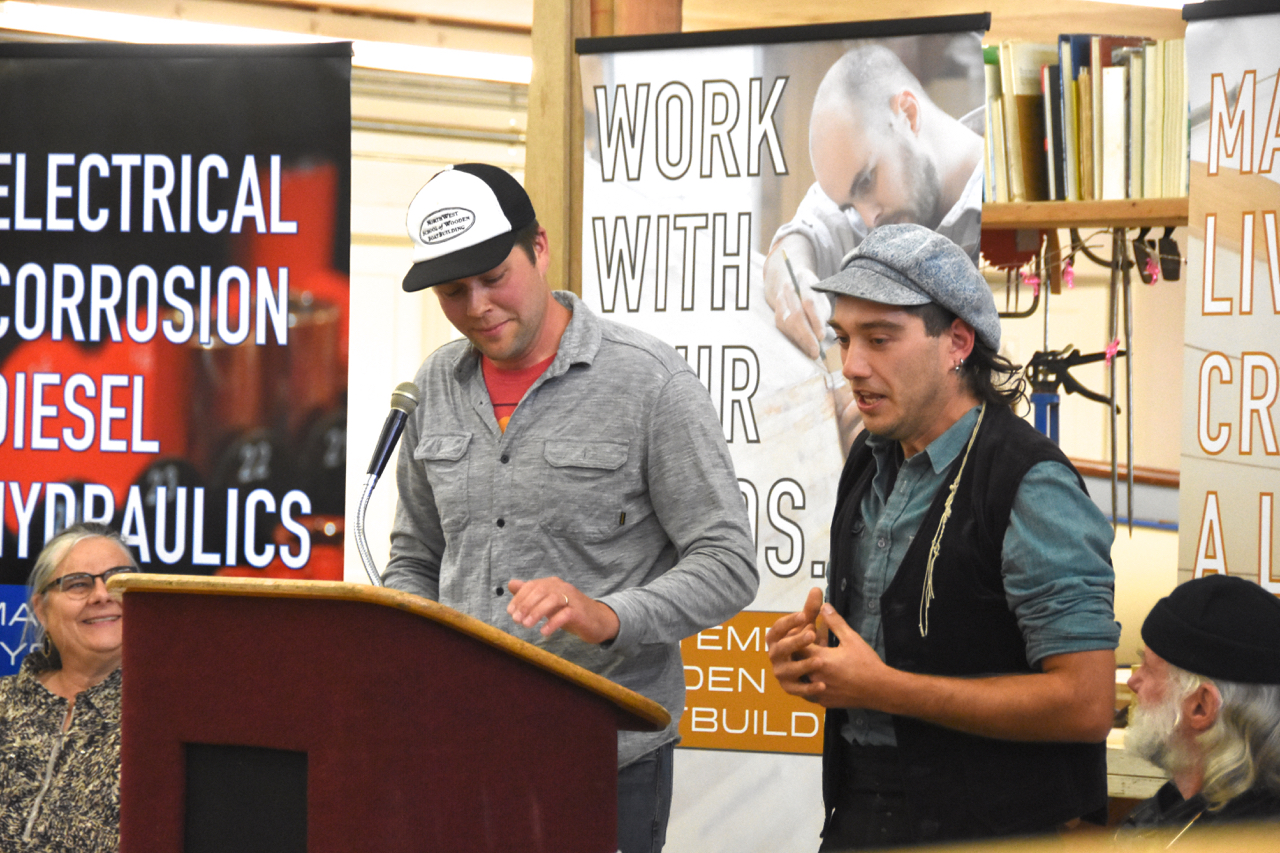The image shows a presentation scene with a wooden podium on the left, equipped with a silver microphone. At the podium, a Caucasian man wearing a black and white baseball cap and a light blue long-sleeve shirt over a pink shirt is looking down at his notes. He is partially obscuring a woman sitting behind him, who is facing the camera. To the right of the man at the podium, another man is speaking. This man has dark hair under a light gray cap, dark eyebrows, and is wearing a blue chambray shirt with a dark vest. He is gesturing with his hands in front of him. Both men appear to be engaged in a presentation, possibly a workshop. In the background, there are large vertical banners with text, though only some words like "electrical corrosion," "diesel," and "hydraulics" are clearly visible. An older woman, smiling, is seated at the bottom left corner, watching the presenters, while an older man with a beard and long white hair, wearing a black knit cap, is in the bottom right corner, also looking towards the presenters. The setting suggests a technical or industrial conference.